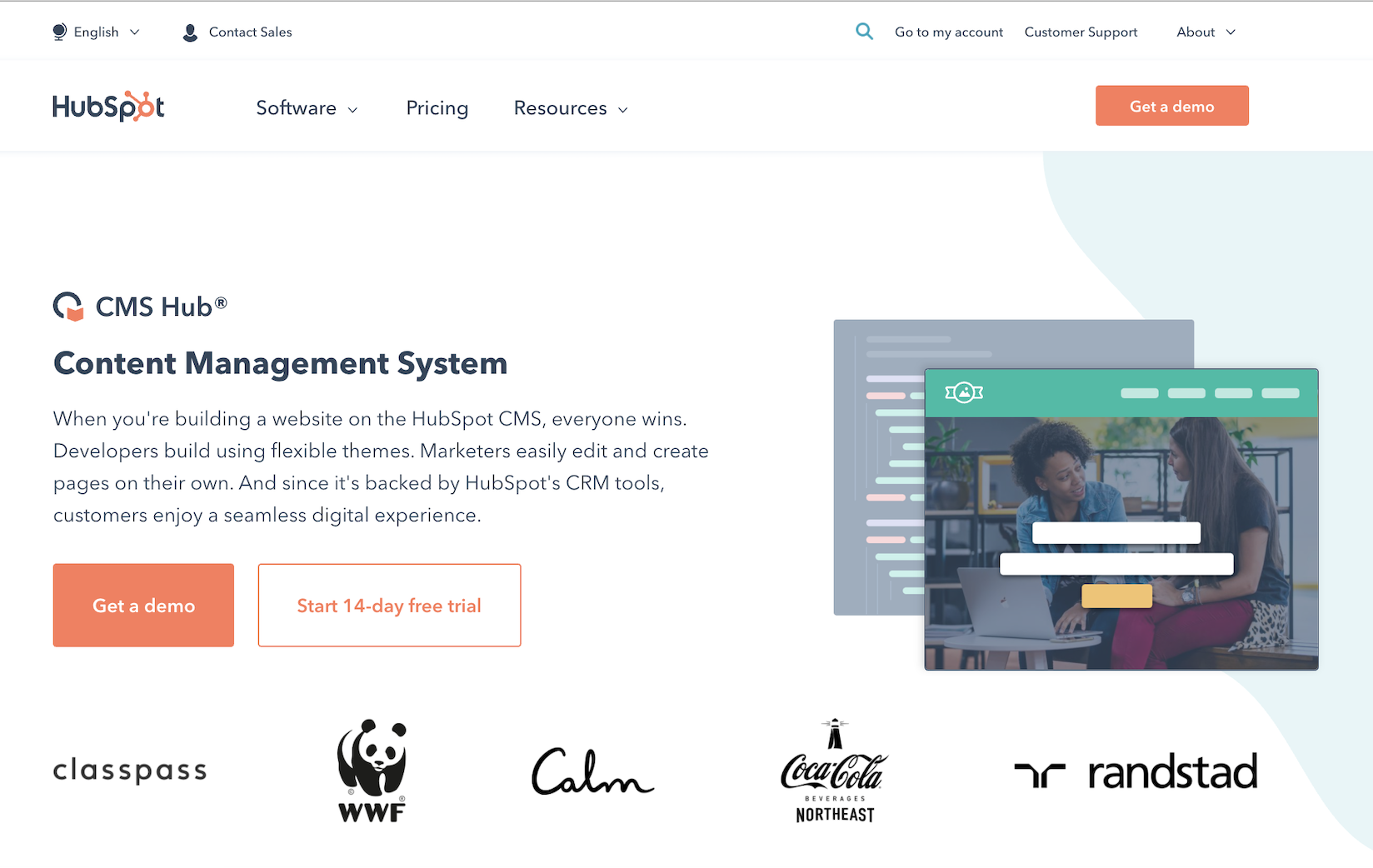This screenshot captures the homepage of the HubSpot website, featuring a clean, white background for a streamlined appearance. At the very top left, there is an English language dropdown menu, accompanied by a "Contact Sales" link. On the top right, a series of links includes a search button, "Go to My Account," "Customer Support," and an "About" dropdown menu.

Below this top navigation bar is the main header. On the far left, the HubSpot logo features prominently, showcasing "HubSpot" in black text with an orange "O." To the right of the logo, a secondary menu includes dropdowns for "Software" and "Resources," as well as a "Pricing" link. This row concludes with an eye-catching orange button labeled "Get a Demo" in white text. 

Beneath these elements, the main content area prominently displays the headline "CMS Hub: Content Management System," followed by a descriptive text passage that extols the system's features and benefits. Continuing down the page, another orange "Get a Demo" button appears, again with white text. Adjacent to this is a white button outlined in orange, with orange text offering a "Start 14-Day Free Trial" option.

This detailed layout underscores HubSpot's user-friendly and fully-featured design, aimed at driving user engagement and highlighting key services.